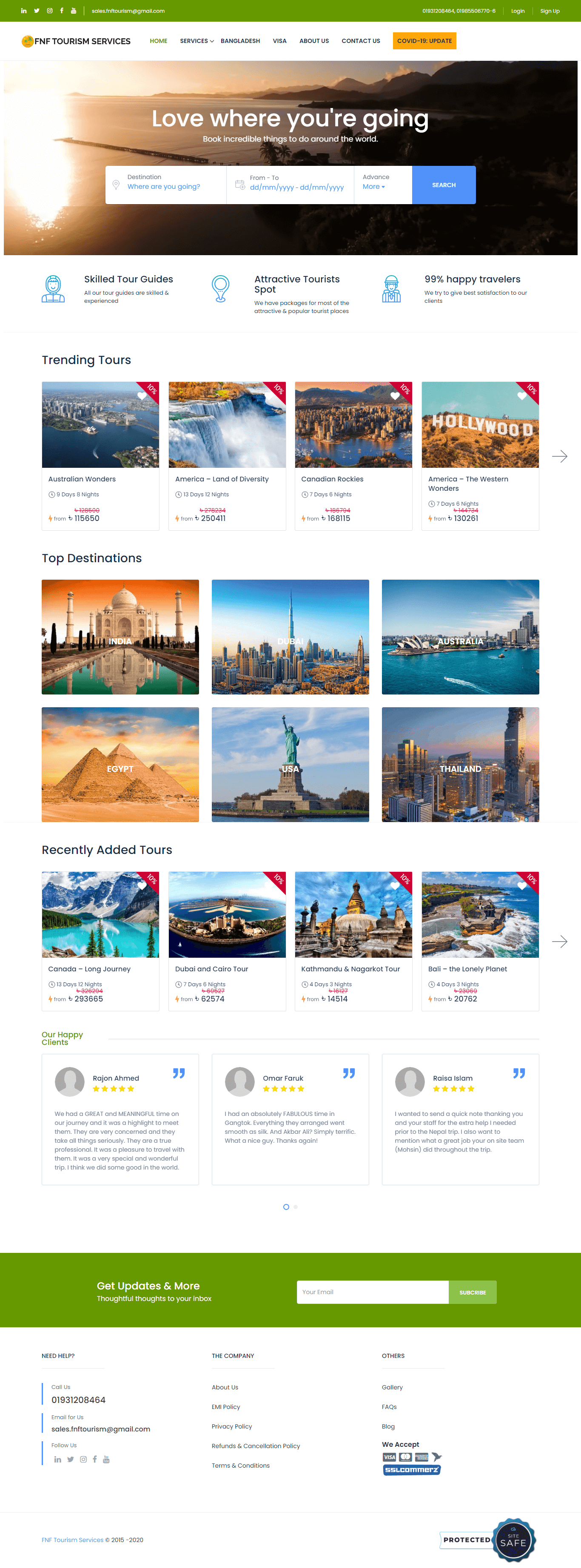### Caption:

This webpage features a clean white background with two prominent green bars—one thin at the top and another thicker at the bottom, both adorned with white text and icons. Despite the clarity of their design, some icons and text are too small to decipher. Beneath the top green bar, there are multiple segments of text wherein the first word is green followed by several black text segments, difficult to read. A yellow bar sits below this text, also with black writing that's hard to distinguish.

Centering the page is an evocative image of a sunset over the ocean, with hills silhouetted on the right, creating a tropical ambiance. The central text on this image, written in white, reads "Love where you're going." Below this image, there's a white search bar with black text inside, alongside a blue box containing the word “Search” in white.

Further down, there's a section titled "Trending Tours" in black. This section showcases four images: a city by the water, a waterfall, oceans with hills, and brown hills featuring the famous Hollywood sign.

The section titled "Top Destinations" follows, presenting two rows of images. The top row includes pictures of the Taj Mahal, the New York City skyline viewed from above, and an aerial shot of an ocean. The bottom row features images of the pyramids, the Statue of Liberty, and another cityscape.

Lastly, under the header "Recently Added Tours," there's a row of four images. These include a photo of water and blue skies, a slightly distorted image of water, what appears to be a stone statue (possibly the Sphinx), and a tropical ocean scene.